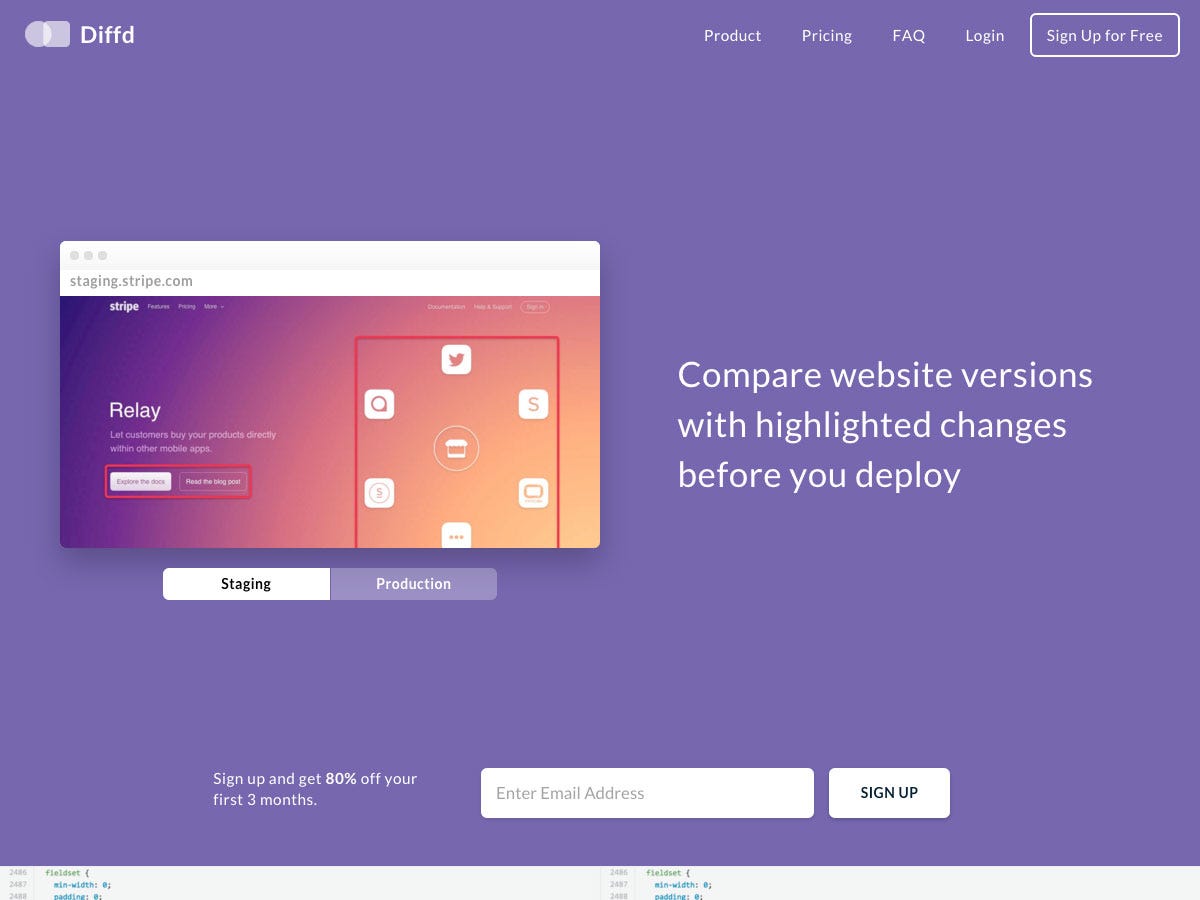This is an image captured from a web page identified as "DIFFD." The overall background is a solid purple color, setting a vibrant tone for the page. At the top of the page, there is a navigation bar with various clickable options. From right to left, the options include: "Product," "Pricing," "FAQ," "Login," and a prominent "Sign Up for Free" button.

On the left side, the text "staging.stripe.com" is visible, likely indicating a development environment for Stripe. Below this, there's a detailed image with icons arranged in a square surrounded by a red outline. The text within the square reads "Relay" and includes a brief description: "Let customers buy your products directly within other mobile apps." Additional text follows with phrases such as "Explore the door" and another partially obscured directive ending with "read."

Further down, there's a section that highlights "staging and production," possibly referring to different operational stages of the platform. A promotional offer states "Sign up and get 80% off your first three months," followed by a field to enter an email address. To the bottom-right of this section, there's a clickable "Sign Up" button designed to prompt user action.